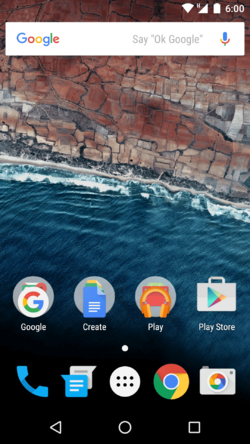The screenshot showcases an Android home screen with various UI elements. At the top right, there are icons indicating Wi-Fi signal strength, cellular signal, battery life, and the current time, which is 6:00. Just below these, there's a Google search bar set against a white background featuring the colorful Google logo. The search bar has the prompt "Say OK Google" and a blue Google microphone icon on the right side.

The wallpaper features a serene nature scene, displaying clear blue water alongside striking orange-red rocks. At the bottom of the screen, there are several app icons including Google, Create, Play, the Play Store, Phone, Messages, the App Drawer, Google Chrome, and the Camera.

Beneath these app icons, there are three navigation buttons: a left-pointing triangle for 'Back,' a circle for 'Home,' and a square for accessing the most recent apps or a secondary menu. These elements collectively provide the key functionalities for navigating the Android operating system.